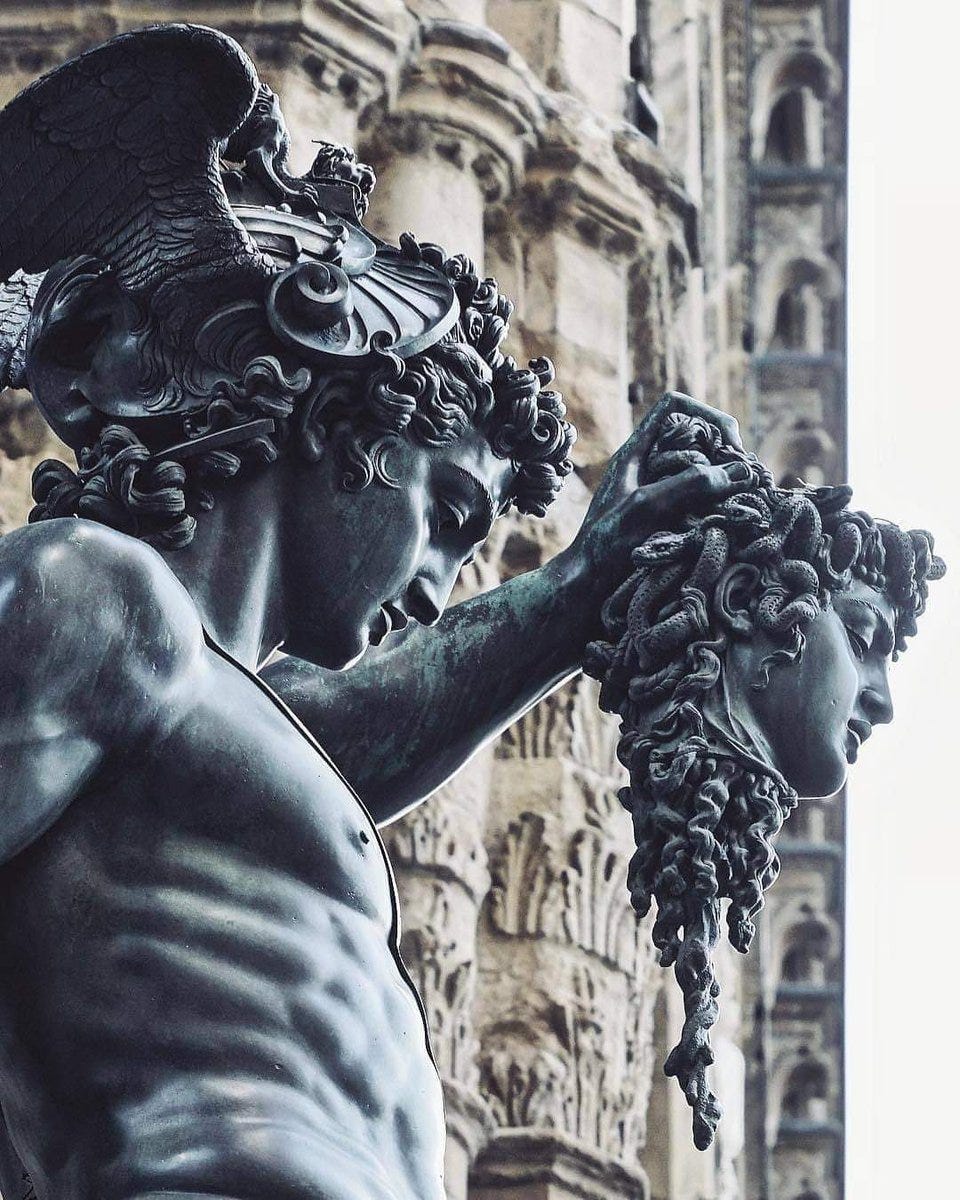In this detailed photograph, a striking statue stands prominently in the foreground against the backdrop of an ornate European cathedral building with tan and beige hues, elaborate columns, and intricate decorations. The statue, which exudes a classical Greek aesthetic, features a young muscular man, his body chiseled with a well-defined six-pack of abs, standing in a slight turn to the right. He is adorned with an elaborate helmet decorated with bird's wings on either side, and his short, curly hair can be seen peeking out from beneath it. The man, resembling the Greek god Mercury, gazes downward with a solemn expression. In his left hand, he holds the severed head of Medusa, easily recognizable by the snakes entwined in place of hair. The gruesome detail of flesh and tendons dangling from her neck adds to the dramatic intensity of the scene. The overall composition, melding the grotesque yet captivating sculpture with the historic and ornate architectural backdrop, creates a powerful and evocative image.